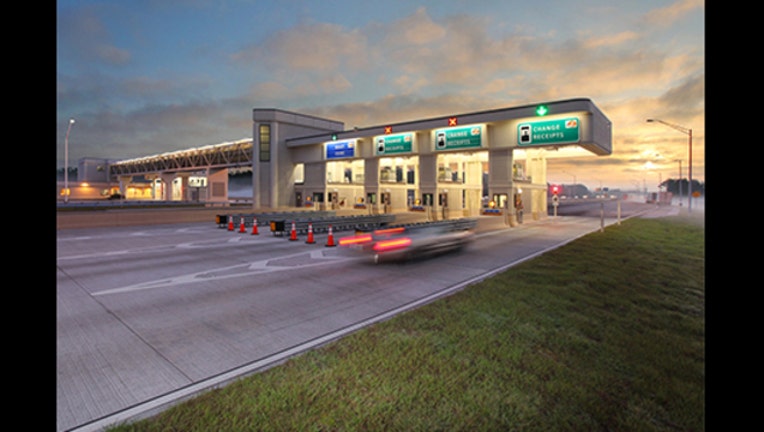The image depicts a border crossing or toll booth with multiple lanes, focusing on four right-hand lanes. The left side of the booth is dark, suggesting it is closed, with cones blocking entry to those lanes. On the right, three lanes display green signs—though two of these lanes have red lights barring entry, while the far-right lane, marked with a green light and green arrow, is open for cars. The third lane from the right has a blue sign. The captured scene shows a car passing through the open lane at high speed, creating a motion blur with red taillight streaks. The setting sun illuminates the sky, indicating it is nearly nighttime. On the image’s far right, a patch of green grass suggests a non-urban setting. The booth has a long roof, and there are black and white striped gates associated with each lane, with some showing red lights indicating closure.